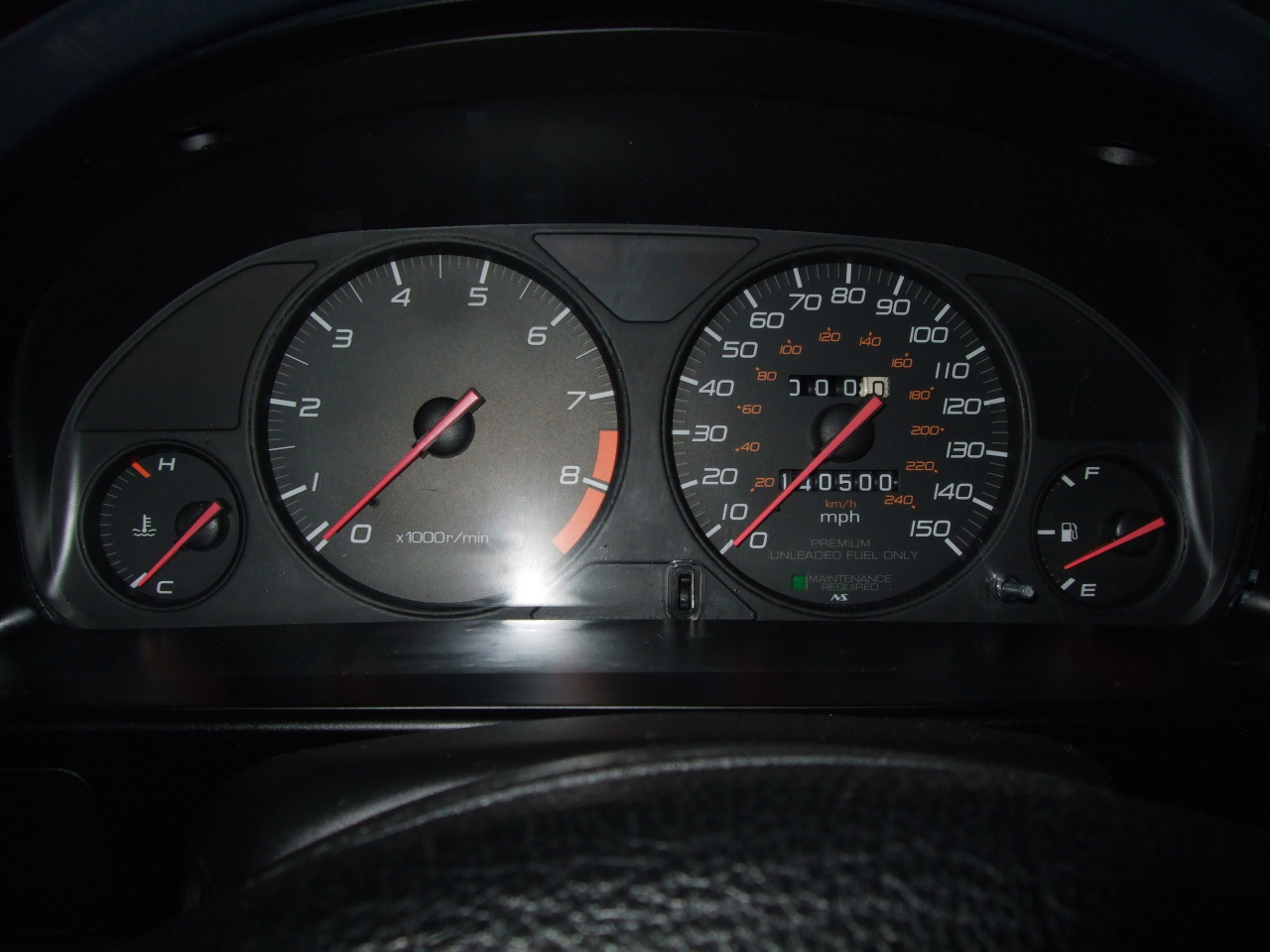The image depicts a detailed view of a car's dashboard, focusing on four essential gauges. In the foreground, a blurred section of the steering wheel can be seen, contrasting with the crisp detail of the dashboard's instruments. The dashboard itself is mostly dark and black, providing a stark backdrop to the bright indicators. 

On the far left, there's a small circular engine temperature gauge with a red needle pointing between "H" (Hot) and "C" (Cold). Next to it is the tachometer, a larger dial with a red needle and a red area indicating high RPMs, labeled "x1000 R per minute" to show engine rotations per minute. 

To the right of the tachometer is the speedometer, marked in miles per hour from 0 to 150, also featuring a red needle, and the kilometers are specifically denoted in orange. Finally, on the far right is the fuel gauge, similar in size to the temperature gauge, with a red needle and the letters "F" and "E" indicating Full and Empty. The entire setup is designed to provide detailed and clear information about the vehicle's status at a glance.